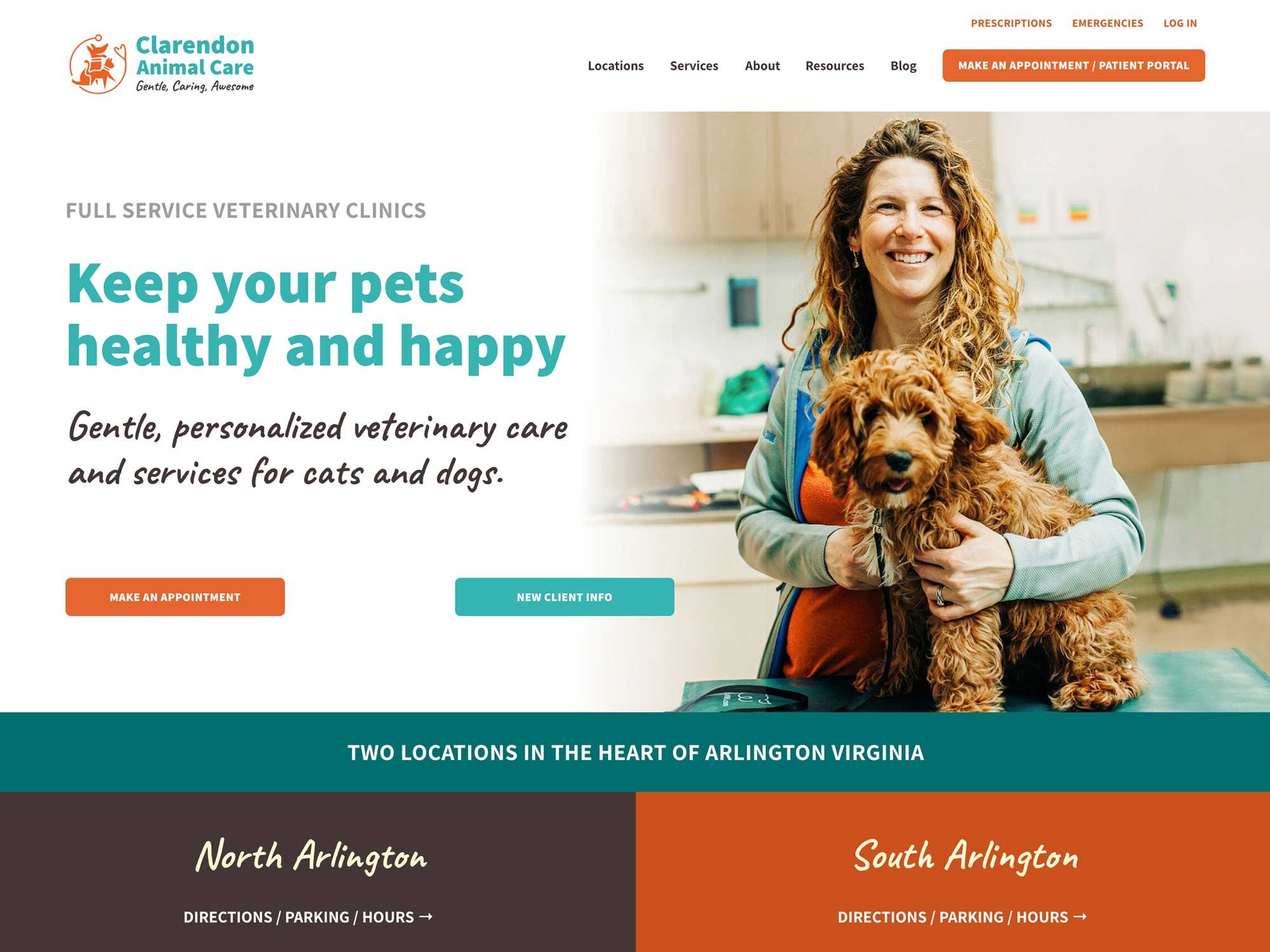This is a detailed caption for an image of a webpage belonging to Clarendon Animal Care:

The screenshot captures the webpage for Clarendon Animal Care, featuring a compact and visually appealing layout. In the top-left corner, an orange logo with a small dog icon is prominently displayed. Adjacent to this logo, the clinic’s name, "Clarendon Animal Care," is written in clean green text. Beneath the name, a line of small black text states "gentle, caring," followed by an unreadable word. To the right, orange text options read "Prescriptions, Emergencies, Log In."

Below this header, the navigation menu in black text includes links to "Locations, Services, About, Resources, Blog." To the right of the navigation menu, an orange button with white text prompts visitors to "Make an Appointment, Patient Portal." 

Further down, the central part of the webpage features an image of a woman standing in a veterinary office with a mid-sized brown dog with longish hair. Next to the image, a block of gray text states, "Full Service Veterinarian Clinics." This is followed by a larger green text declaring, "Keep Your Pets Healthy and Happy." Complementing this, a handwritten-style black font reads, "Gentle personalized veterinary care and services for cats and dogs." 

Positioned below this text are two call-to-action buttons: an orange one labeled "Make an Appointment" and a green one labeled "New Client Info." 

A green banner beneath these buttons highlights "Two locations in the heart of Arlington, Virginia." This section is bifurcated into a black section for "North Arlington" and an orange section for "South Arlington," each listing "Directions, Parking and Hours" below.